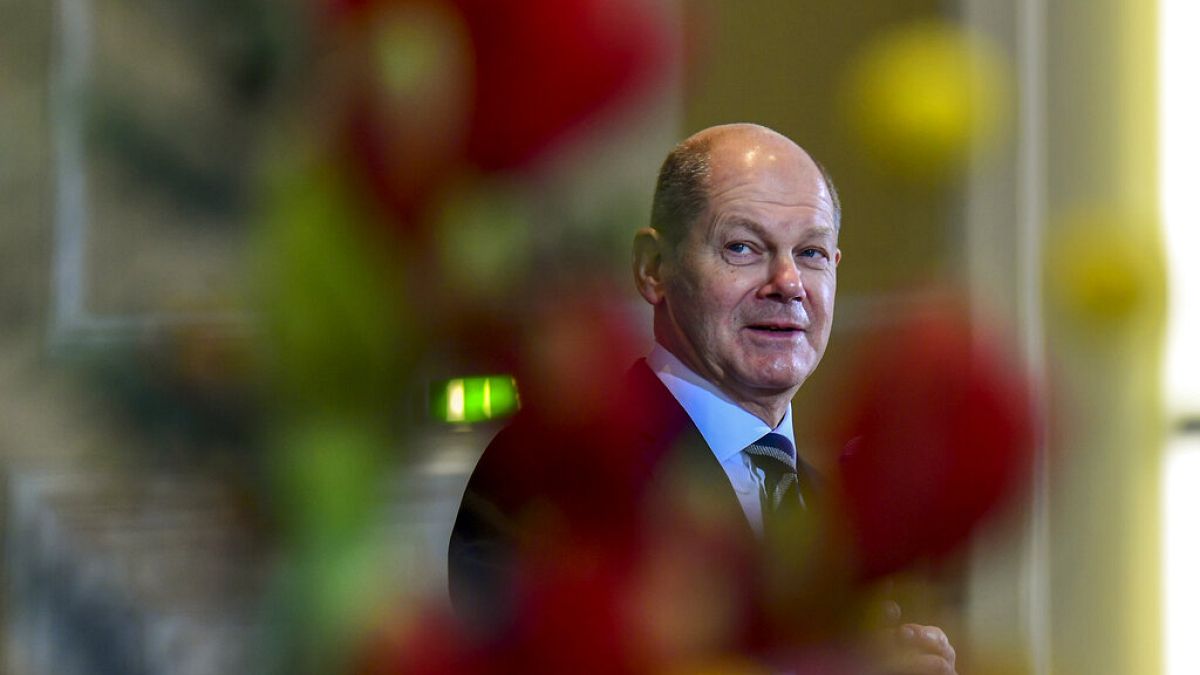This color photograph captures an older white man roughly in his seventies, positioned just right of center in the frame. He has a bald head with short gray hair on the sides. He's dressed in a dark blue suit, a white or light blue button-down shirt, and a striped tie featuring blue and gray hues. The man's body is angled to the right, but his head is turned forward with his eyes gazing toward the left of the frame, displaying a dubious or somewhat amused expression. His mouth is slightly open. In the foreground, there is a blurry, out-of-focus element resembling leaves or foliage, possibly from a potted plant or a bouquet of red roses, creating the effect of him being viewed through greenery. The background features the painted walls and wood paneling of an interior setting, suggesting the indoor environment. Additionally, there are white frames, and what appears to be a fireplace, adding further context to the room's décor.